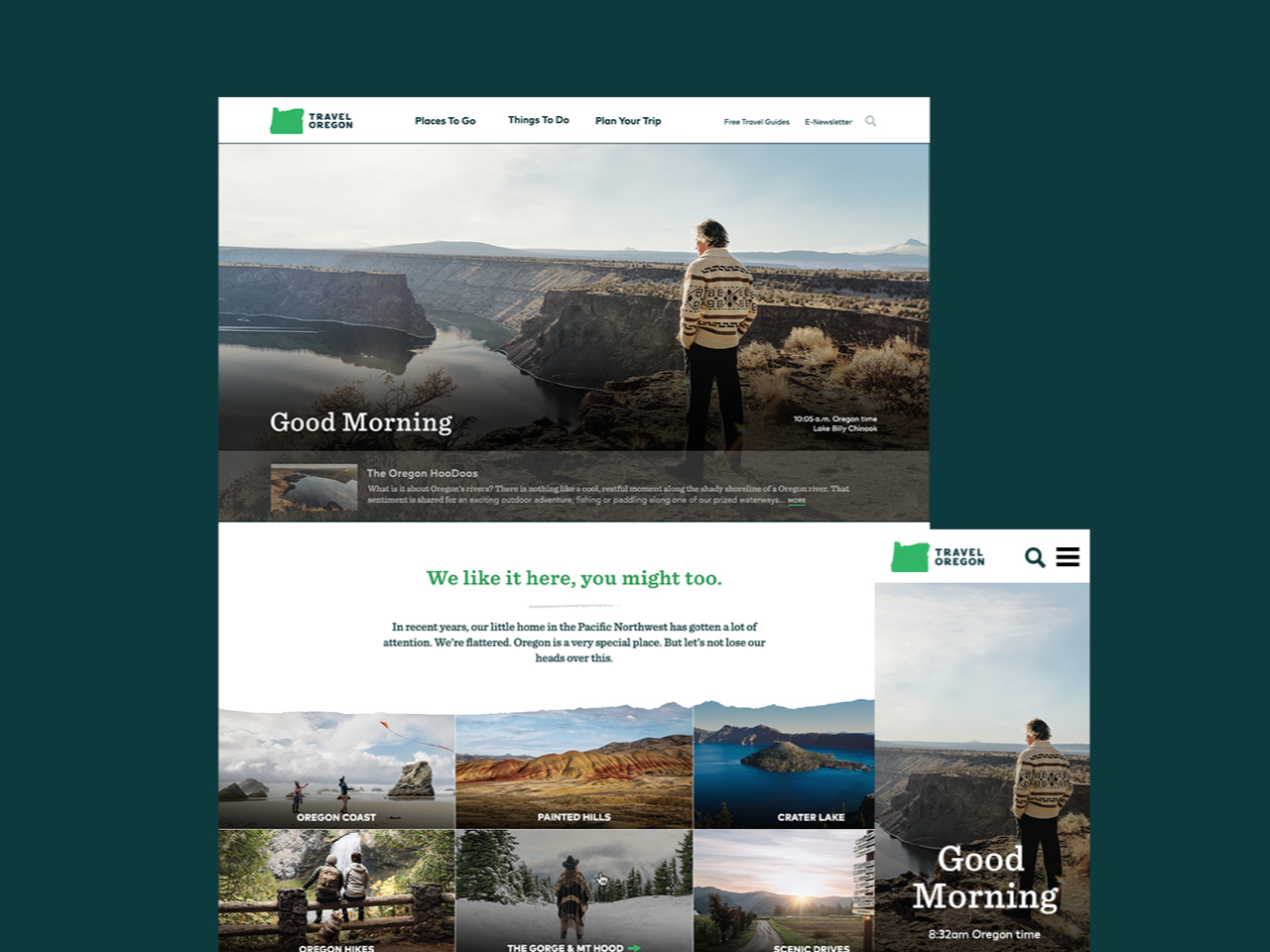A meticulously crafted collage showcases a couple of web pages against a rich, deep greenish-bluish-gray background, presenting a snapshot of the "Travel Oregon" website. At the top, the main section prominently displays "Travel Oregon" beside a green silhouette of the state of Oregon. Below this header, navigational options are displayed, including "Places to Go," "Things to Do," "Plan Your Trip," "Free Travel Guide," and "E-Newsletter."

Within the image, a man in a patterned sweater gazes thoughtfully over a picturesque gorge river area, accompanied by the welcoming message "Good Morning." Below him, the website introduces "The Oregon 'Who Do's" along with some informational text.

Following this, a subsequent section captures attention with a green header reading, "We like it here. You might too." This part elaborates, explaining that Oregon, a gem in the Pacific Northwest, has garnered significant attention in recent years, earning flattering recognition without succumbing to arrogance.

Additionally, the page highlights various Oregon attractions such as the Oregon Coast, Painted Hills, Crater Lake, Oregon Hikes, the Gorge, and Mount Hood. Each attraction is paired with a visual, inviting explorers to delve into the scenic beauty and diverse adventures awaiting in this extraordinary state.